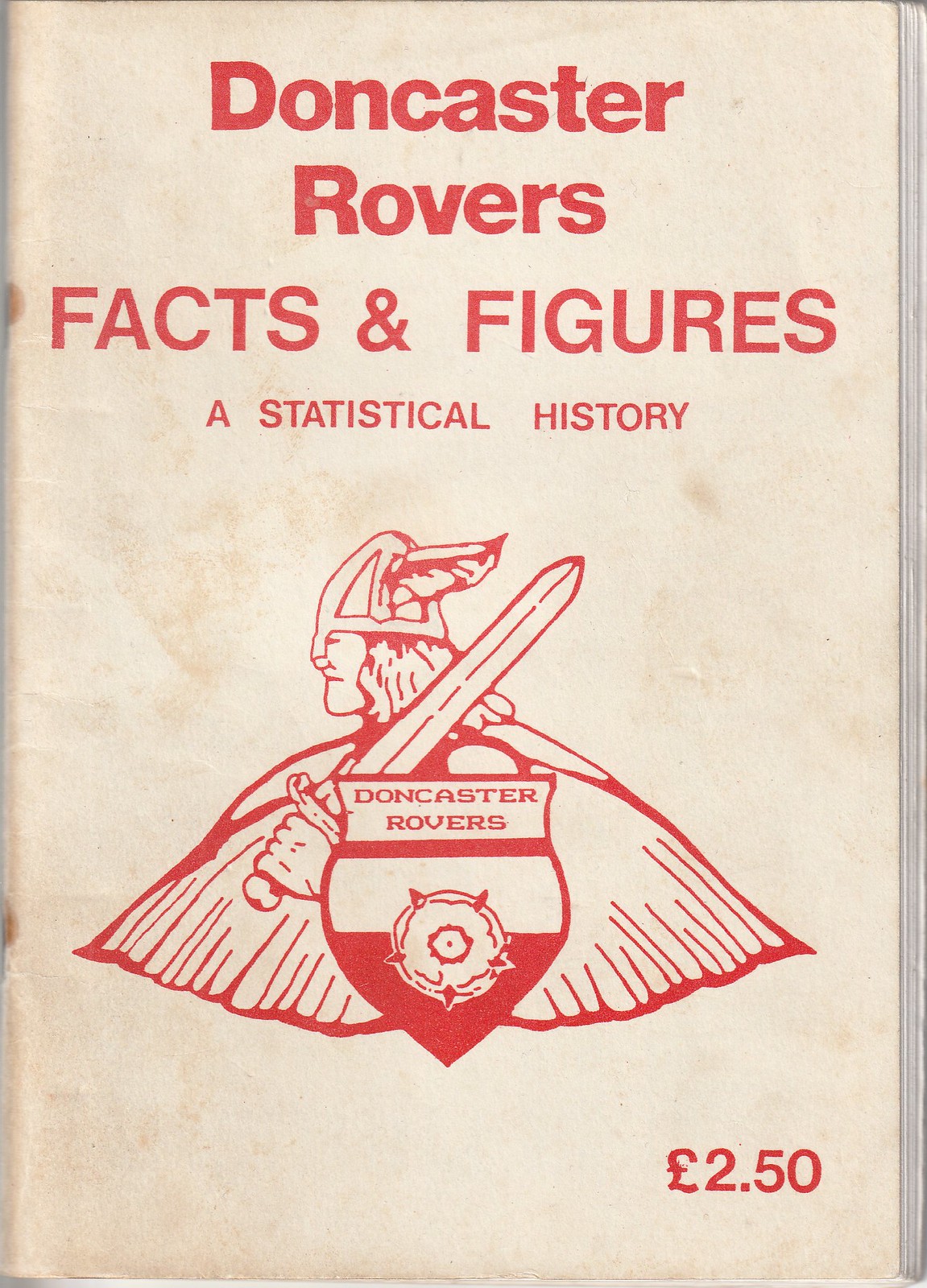The image depicts the front cover of a vintage, scanned booklet titled "Doncaster Rovers Facts and Figures of Statistical History." The background is a beige off-white or tan stock with a pebbled or patchy texture, accented by dirt marks and a noticeable stain on the bottom left. The title is prominently displayed in bold red font, with "Doncaster Rovers" at the top and "Facts and Figures of Statistical History" in uppercase, smaller print just below.

In the lower portion of the cover, there's a red insignia featuring a warrior in profile facing left, wearing a winged Viking helmet and brandishing a broadsword in the left hand. The warrior stands behind a shield inscribed with "Doncaster Rovers." The booklet, which appears to be held together by staples, is priced at 2 pounds 50, indicated in the bottom right corner. The overall dimensions suggest a small, rectangular booklet designed to provide historical statistics, likely related to the Doncaster Rovers soccer team.